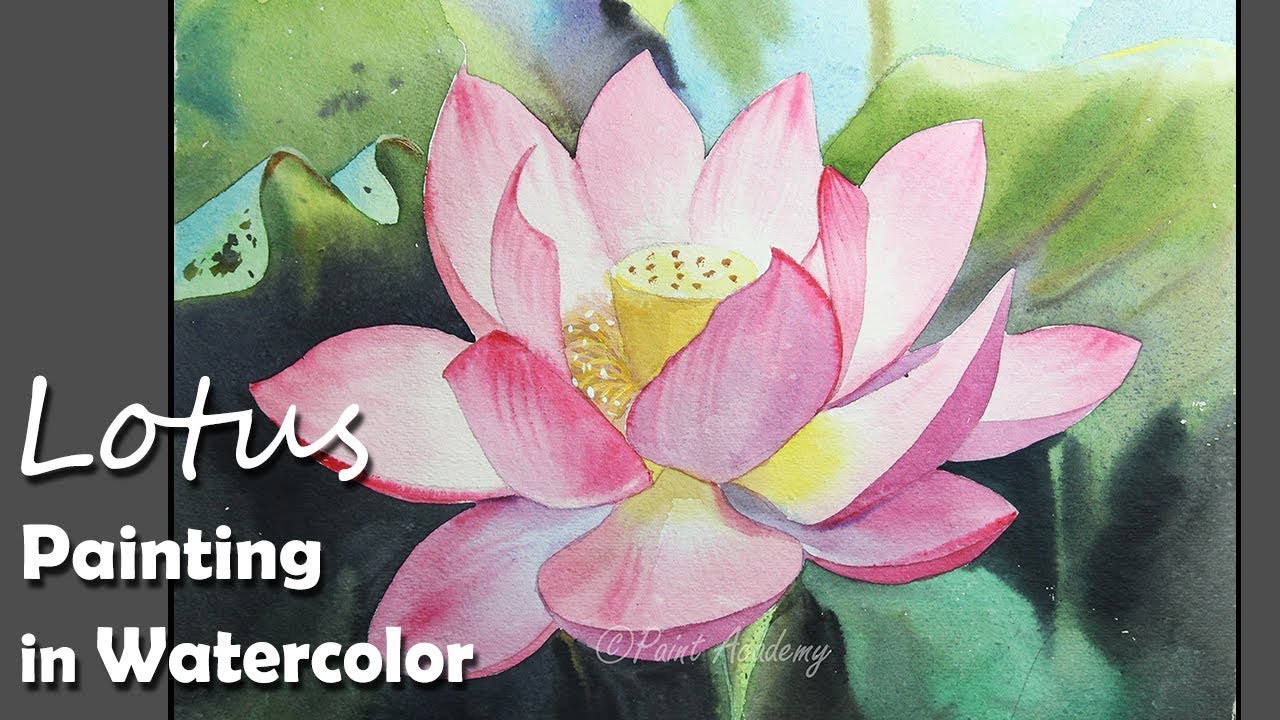This is a high-quality photograph of a vibrant watercolor painting of a lotus in various shades of pink and purplish hues. The lotus is depicted with half-opened petals, showcasing a yellow core with little spots. The stem is vividly yellow. Surrounding the bloom, there is an array of green leaves, ranging from seafoam green to darker shades, with one large leaf draping over the top left edge like a flag. The background features a mix of blue and black tones, giving a subtle contrast to the sharply painted blossom. The image also includes text in white to the left, stating "Lotus, Painting in Watercolor," with "Lotus" in a different font. Lower on the image, a small watermark reads "Copyright Paint Academy," reinforcing its artistic authenticity. The composition has a balance of bright colors and softer, less defined green and black elements, possibly representing lily pads.